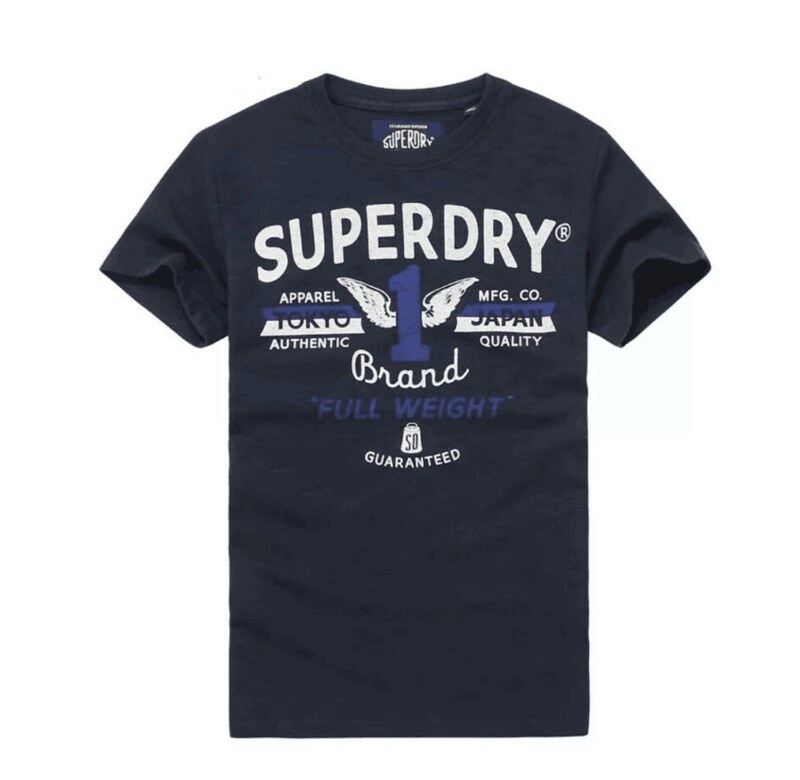The image depicts a black graphic t-shirt prominently displayed against a solid white background. The shirt features a detailed design with large, bold white text at the top that reads "Superdry." Below this, a blue number "1" with white wings extends outwards. Flanking the wings, the text reads "Apparel Tokyo Authentic" on the left side and "MFG Co. Japan Quality" on the right. Centered beneath the number "1" is the word "Brand" in cursive white text. Below "Brand," in a lighter blue shade, the words "Full Weight" are displayed. Further down, a white icon resembling a weight is positioned with the letters "SD" above it and the word "Guaranteed" at the very bottom. Additionally, the tag inside the neckline confirms the shirt is by Superdry.